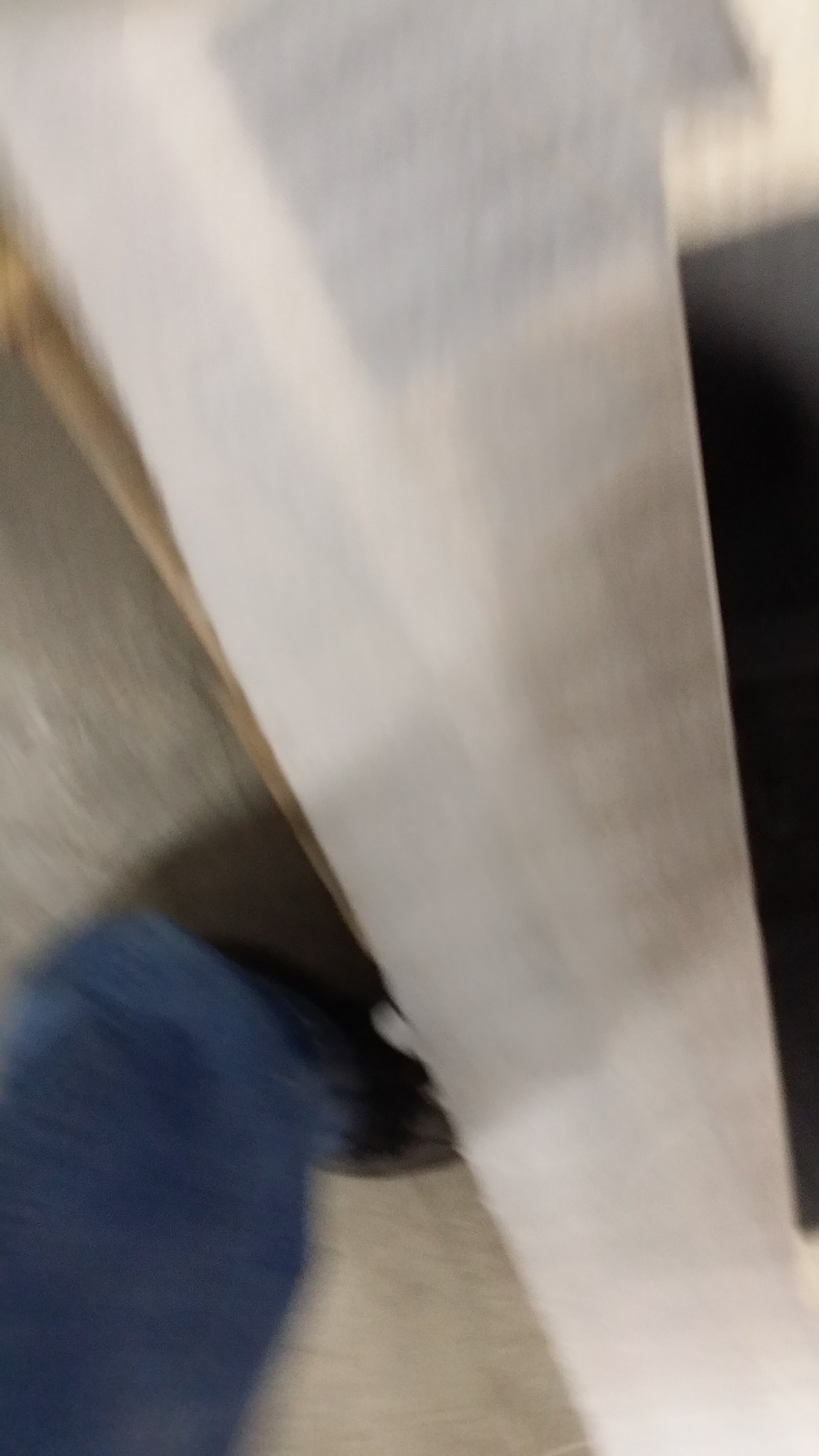The image is quite blurry, but it appears to capture a scene dominated by a striking white beam that diagonally stretches from the bottom right corner towards the top left corner. The beam extends horizontally near the top, reaching almost to the right edge before stopping about half an inch short. The area opposite the beam is predominantly dark. On the left side of the beam, a person's leg is visible, clad in blue jeans and a dark-colored sneaker. The neutral-colored floor beneath the leg features a shadow cast by the person, situated close to the sneaker.